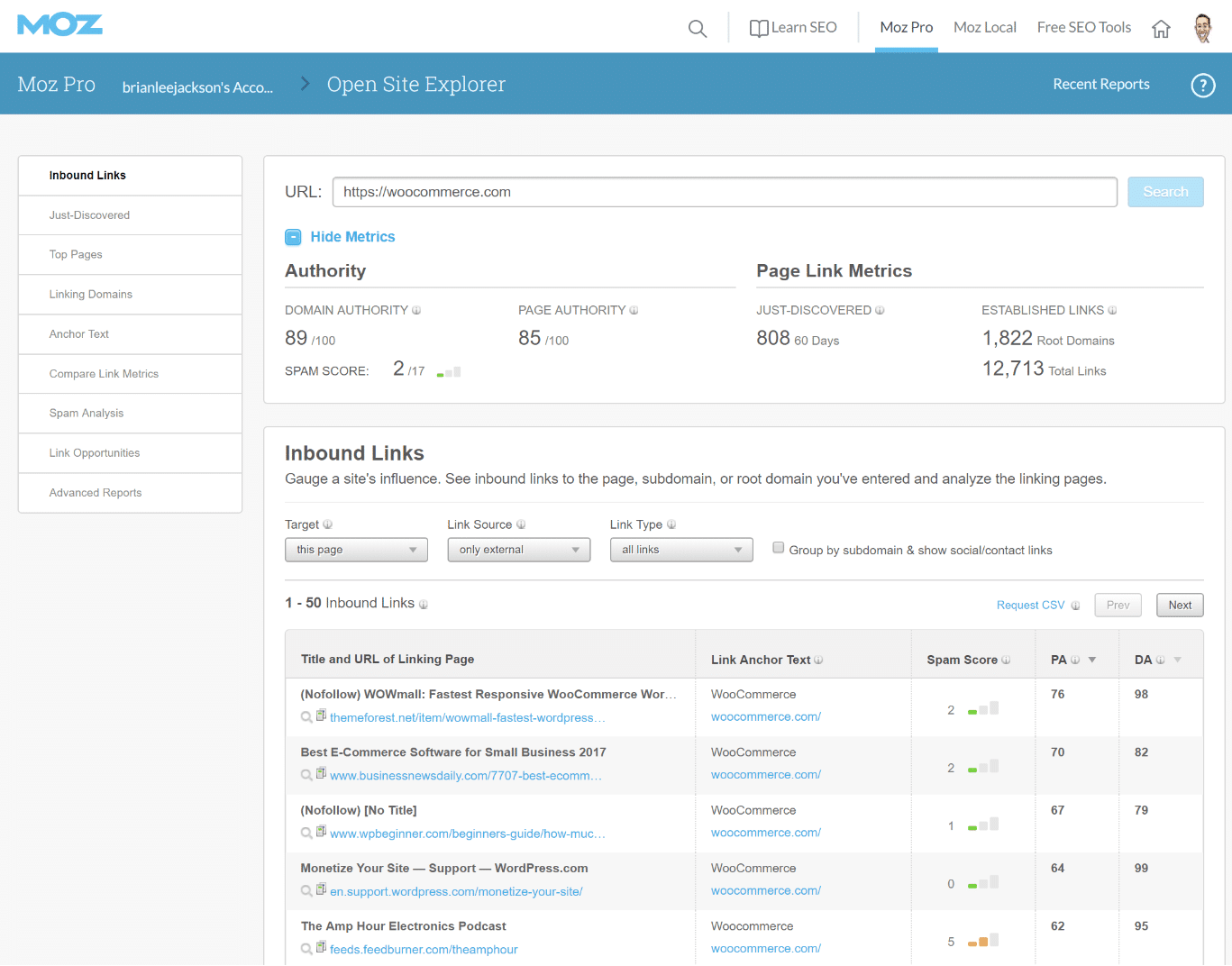In this image, we see an opened webpage from Moz, characterized by its distinct blue and white color scheme. At the top of the page, the brand name "Moz" stands out in blue against the white background. On the top right, a navigation menu includes icons and links for "Search," "Learn SEO," "MozPro," "MozLocal," "Free SEO Tools," and "Home," along with a user profile.

Directly below the navigation menu, we see details pertaining to a MozPro account belonging to "Brainly Jackson." The section features various options such as "Open," "Science Explorer," and "Recent Reports," set against a blue background with white text.

Further down on the right side, there’s an extensive list related to inbound links. This list includes categories like "Just Discovered," "Top Pages," "Linked Domains," "Anchor Texts," "Compile Links," "Metrics," "Spam Analysis," "Link Opportunities," and "Advanced Reports." Adjacent to this list, under a section labeled "URL," the website WooCommerce.com is displayed within a search bar.

Key metrics for WooCommerce.com are shown, including:
- **Height Metrics** highlighted in blue
- **Authority and Domain Authority:** 89 out of 100
- **Page Authority:** 85 out of 100
- **Spam Score:** 2 out of 17

The "Page Link Metrics" section details:
- **Just Discovered:** 808 links in the last 60 days
- **Established Links:** 1822
- **Robot Root Domain:** 12713 total links

At the bottom, the "Inbound Links" section indicates the page’s influence, offering detailed insight into the inbound links pointing to the specified page, subdomains, or root domain. Users can analyze these linking pages based on different criteria.

This comprehensive layout provides a detailed view of the site's link metrics and SEO performance, useful for marketers and analysts.